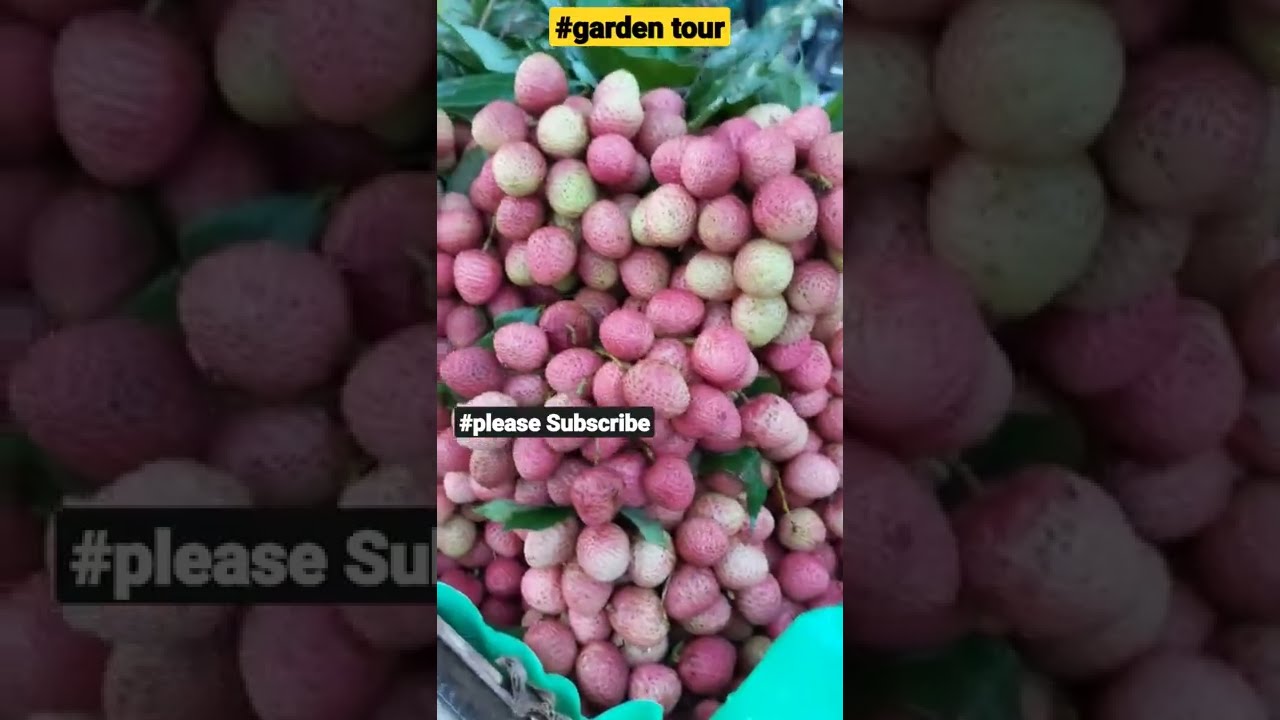The image showcases a bunch of small, pinkish-yellow fruits, possibly an unfamiliar type of berry, with a few green leaves sticking out, arranged in what appears to be a basket or container. The container seems lined with a foam or teal-colored protective pad. The middle section of the image, taking up about one-third of the space, prominently features these fruits. Above this section, there's a yellow box with black text reading "#garden tour". Additionally, towards the lower right side, there is another black text box with white text saying "#please subscribe". The left and right sides of the image consist of blown-up, semi-transparent versions of the same central image, creating an interesting background effect. This design seems to help fill the photo space creatively.